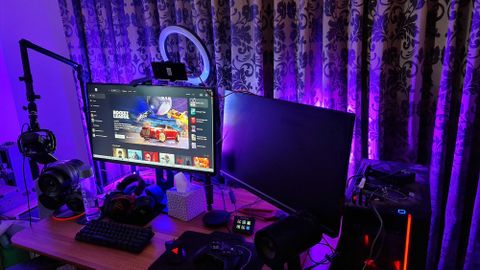The image depicts a dimly lit room, possibly a home office, illuminated predominantly in a vibrant purple hue. Central to the scene is a small brown desk featuring dual computer monitors. The left monitor displays a website resembling Netflix, showcasing TV show recommendations, while the right screen remains blank. Behind the screens, a ring light is positioned to illuminate the user’s face during use. A variety of items scatter the desk: a box of tissues, a headset, an indistinct game controller, and multiple keyboards—though many of these items blend into the shadows due to the backlighting. The backdrop of this setup includes curtains with a subtle floral pattern, accentuated by the room's purple glow. Additional colorful objects—hints of orange, blue, black, white, yellow, and red—dot the scene, though their details are obscured by the lighting and shadows.